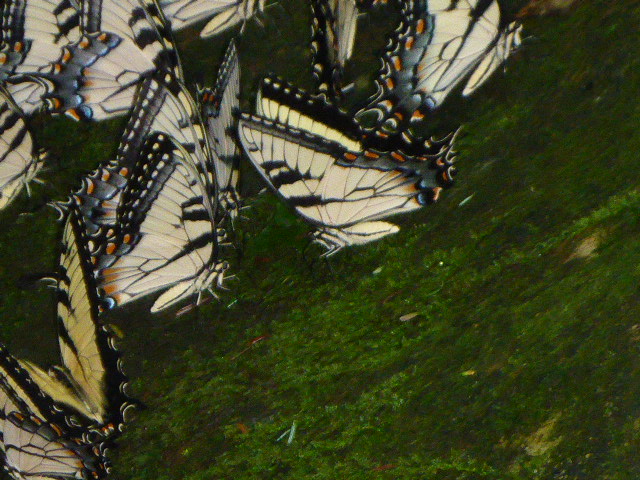The image features a close-up of around seven or eight butterflies resting on a vibrant, mossy surface that dominates the entire background. If you were to draw a diagonal line from the upper right to the bottom left corner, the butterflies are mostly clustered in the upper half above the diagonal. The butterflies are predominantly white, adorned with intricate black outlines, and delicate black veins running through their wings. Some butterflies also exhibit hints of blue and orange near the wing tips. Their bodies are white with a slender black stripe running from head to tail. Most of the butterflies are facing to the right, with a few facing left, and they appear to be either resting or communicating. The mossy surface provides a lush green setting, though some descriptions suggest the presence of very healthy and short grass. The image is captured in sharp detail, highlighting the delicate features of the butterflies, although there is a slight blur that lends a sense of motion to the scene.